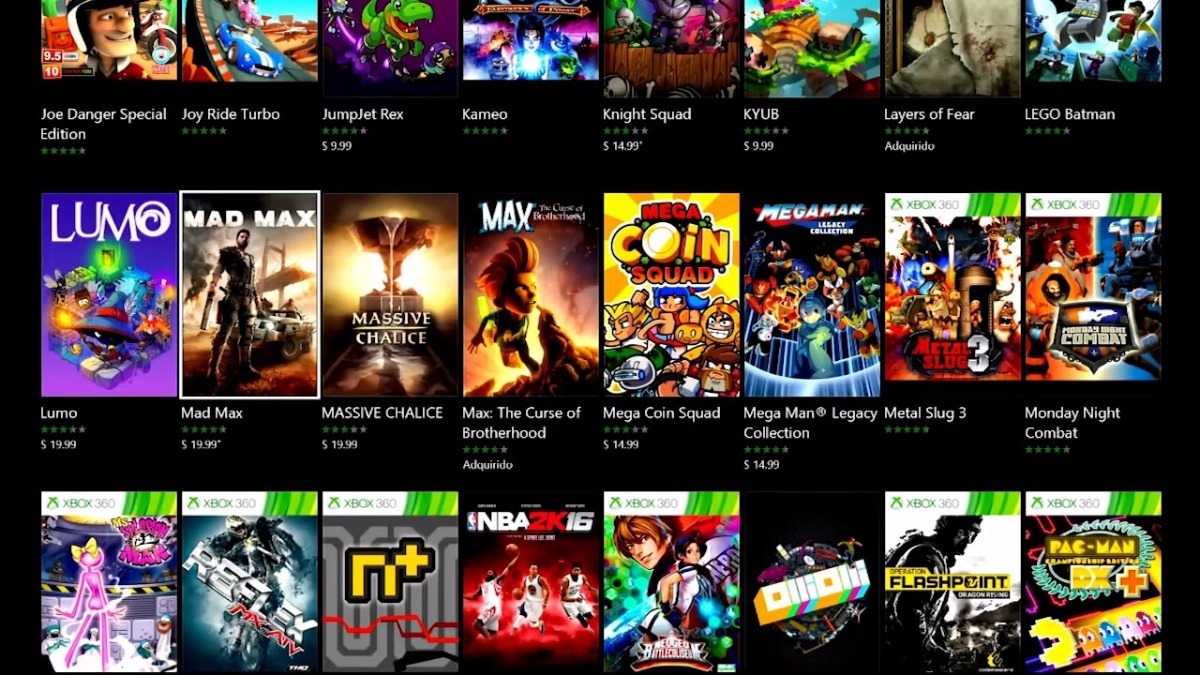This image showcases a curated selection of video games available for purchase, depicted in a clean, organized layout. The games are arranged in three rows, each featuring rectangular images that represent the respective games. Below each image, the name of the game is displayed in white text, accompanied by a star rating and the price.

In the second row, the first game is titled "Lumo." The game's cover art features a mystical setting with glowing green objects intertwined with yellow and blue elements, set against a vibrant purple background. Notably, the letter 'O' in "Lumo" is artistically swirled, adding a whimsical touch.

Adjacent to "Lumo" is the game "Mad Max." The cover illustrates a post-apocalyptic scene with a burning bridge and a gritty atmosphere. A military-style vehicle is depicted, along with a rugged man wielding a weapon in his left hand, dressed in a desert army outfit. The background features multiple fires, emphasizing the chaotic environment of the game.

Further to the right is "Max: The Curse of the Brotherhood." The cover features a dynamic cartoon character with high, reddish-golden hair that curls backward dramatically. He appears to be leaping away from a mountain, with his right hand and fingers clearly visible, while his left hand is clenched into a fist in front of him, portraying an action-packed moment.

This detailed layout not only highlights various games like "Lumo," "Mad Max," and "Max: The Curse of the Brotherhood" but also provides essential information like ratings and prices to assist potential buyers in making informed decisions.